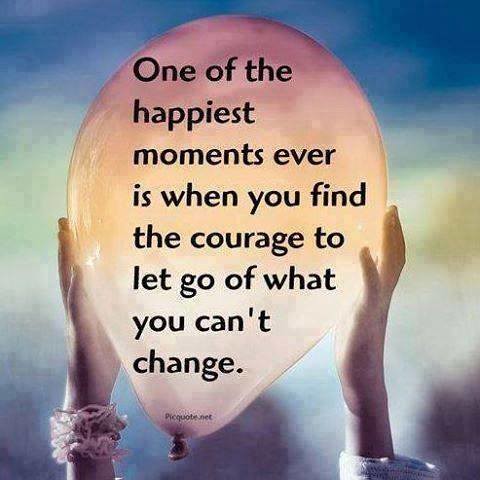This inspirational poster features a large, light orange balloon with a soft gradient that darkens to purplish hues at the top. The balloon is held aloft by two small hands, suggesting those of a young child. The right hand shows a shirt cuff while the left hand is adorned with a unique, interconnected mesh of colorful yarn bracelets. Black text is elegantly inscribed vertically down the balloon, reading: "One of the happiest moments ever is when you find the courage to let go of what you can't change." The background provides a whimsical, painterly effect with horizontal streaks of blue at the top, transitioning through green and yellow, and culminating in a deep purple at the bottom.